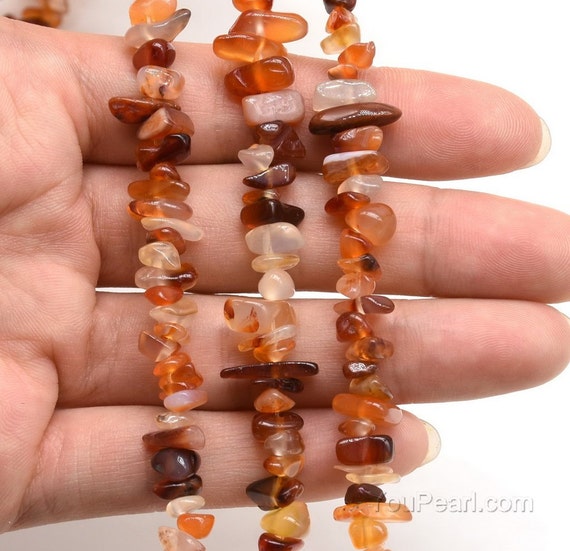This close-up photograph captures a white woman's hand emerging from the left, fingers extended to the right, with three vertical strands of pebble necklaces draped across her outstretched fingers. The necklaces, intricately beaded with a variety of smooth and polished stones, include hues of orange, clear, white, light brown, and dark brown. Each strand runs parallel over her fingers, displaying an array of tiny, flat rectangular to curvy pebble-like stones. The background is a clean, solid white, emphasizing the subtle watermark in the bottom right corner that reads "youpearl.com" in a very light gray font.